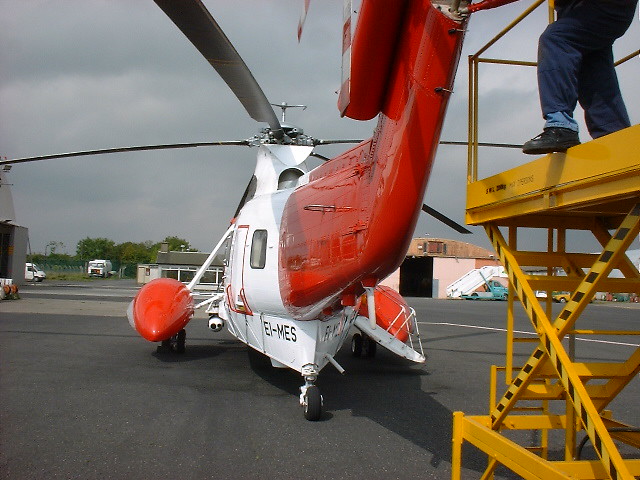This is a detailed color photograph in landscape orientation, capturing the rear view of a helicopter as seen from the tarmac. The helicopter's body features a striking combination of bright red and shiny white colors, with the back half and tail in red and the front end in white. It has very long, stationary blades, with five propellers overhead. The helicopter is equipped with pontoons on each side, finished in a glossy orange and conically shaped, which support the main gear.

A prominent feature in the foreground is a yellow metal extension ladder in an upright position, positioned to the right side of the image. At the top of this ladder is a worker, whose legs are visible, dressed in dark pants and shoes, apparently engaged in maintenance work on the tail rotor. This rotor is associated with a Sea King type helicopter, known for its use by the Navy for rescuing pilots at sea.

In the background, several structures and vehicles are visible. To the right of the image is a hangar with an open door, in front of which is a stair truck. Another hangar is visible to the left, partially cropped by the image. The overall setting is an airfield with several parked vehicles scattered along the tarmac under a gray, cloudy sky, contributing to a representational realism style of photography. A closer inspection reveals a gimbal camera situated between the left-side pontoon and the helicopter fuselage, adding to the helicopter's complex equipment. Toward the bottom of the tail, the marking "E-I-M-E-S" is visible near the tail wheel.